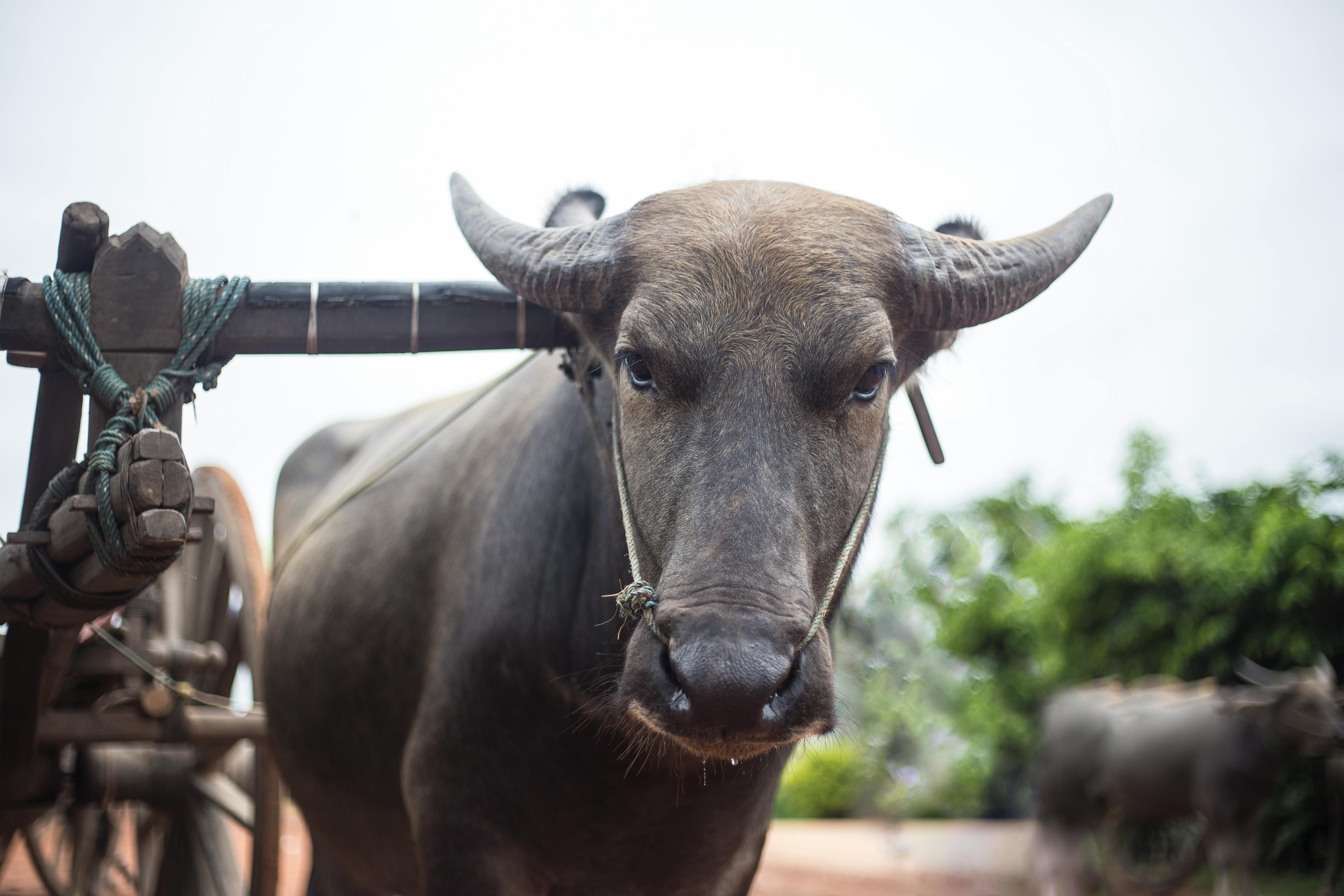This outdoor photograph captures a farm-like setting featuring a scene rich in detail and motion. Central to the image is a sturdy bull, colored in shades of brown and black, with pronounced horns pointing upwards. The bull’s nose is pierced by a rope, which leads back to a wooden bullock cart hitched behind it. The bull's body is fully visible, though the legs are obscured. To the bottom left of the frame, part of the wooden cart is prominently positioned and appears to be designed for transporting heavy loads. This cart is connected to the central bull. In the right background, there is another bull and some green trees, albeit blurred, adding depth to the scene. Complementing the earthy tones are the colors gray, brown, green, and orange, providing a natural palette. Above, the sky transitions from light blue at the sides to white towards the center, contributing to a serene yet industrious atmosphere. There is no text on the image, ensuring that the viewer’s focus remains on the vivid farm scenery and the details within it.